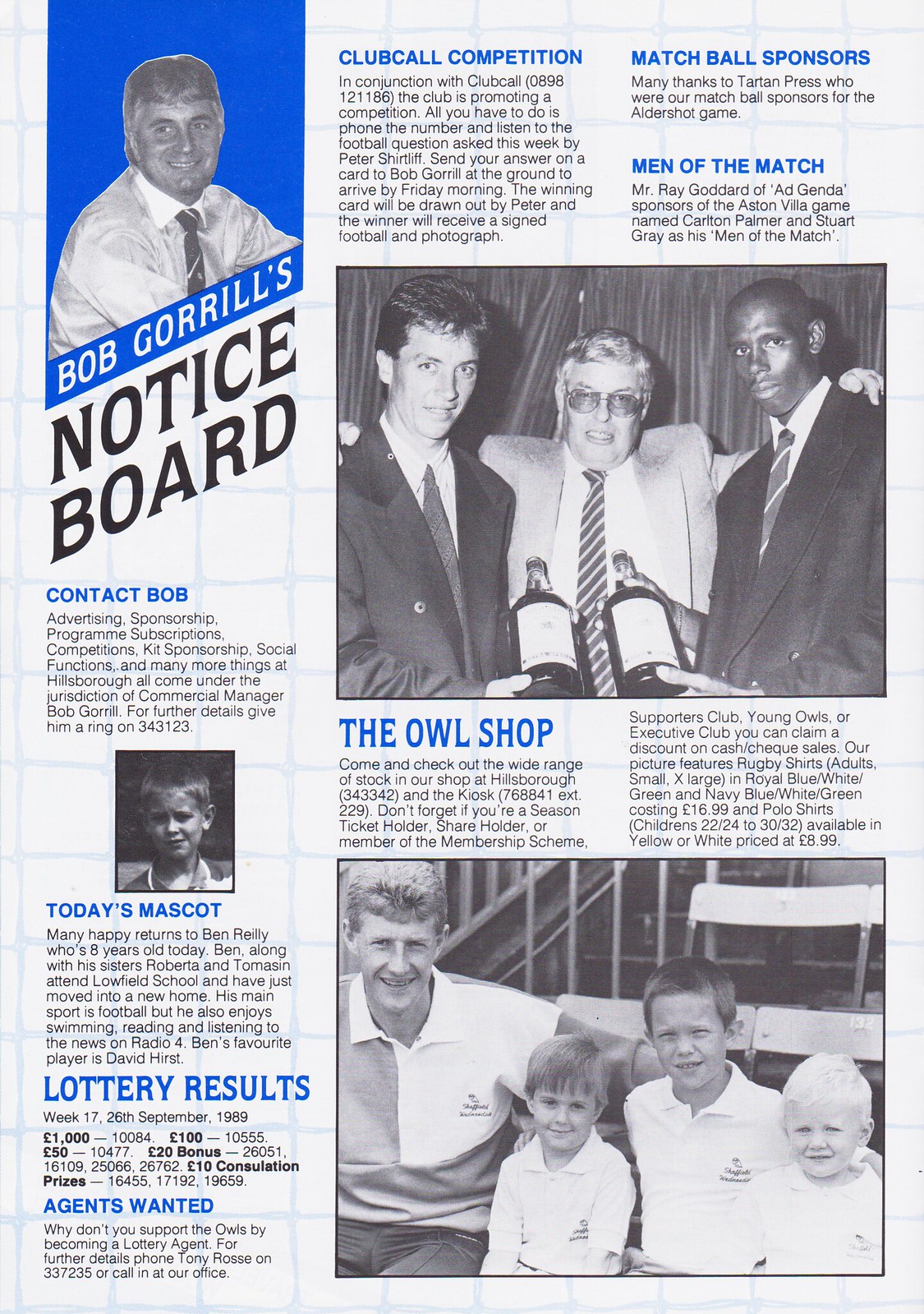This image appears to be a page from an old magazine, program, or brochure, featuring a detailed layout of a notice board. The background is predominantly white, adorned with a subtle light blue grid creating a square pattern. Dominating the top left section is a black and white photograph of an older Caucasian man wearing a tie, positioned slightly angled as if at the five o'clock position, set against a medium blue backdrop. This section is captioned with "Bob Grills Notice Board," though variations of the surname are noted.

Below this photograph, there's contact information for Bob, followed by a series of sections and articles. Key headings include “Today's Mascot,” “Lottery Results,” “Agents Wanted,” “Club Call Competition,” “Match Bill Sponsors,” and a highlighted feature, “Men of the Match,” accompanied by a photograph of the men in question.

On the right side of the page, two distinct black and white photographs are printed. The first image shows two young men holding large bottles of wine or champagne, with an older man in tinted glasses and a sports coat posing with his arms around them. Below this, the text "The Owl Shop" introduces another photograph, this time of a family group that appears to consist of a father and three children, all donning logo-emblazoned shirts likely associated with The Owl Shop or possibly the sports club featured.

Overall, the page merges multiple visual elements, extensive text, and a classic editorial style to present a well-rounded, information-rich notice board meant to engage readers with various announcements and community highlights.